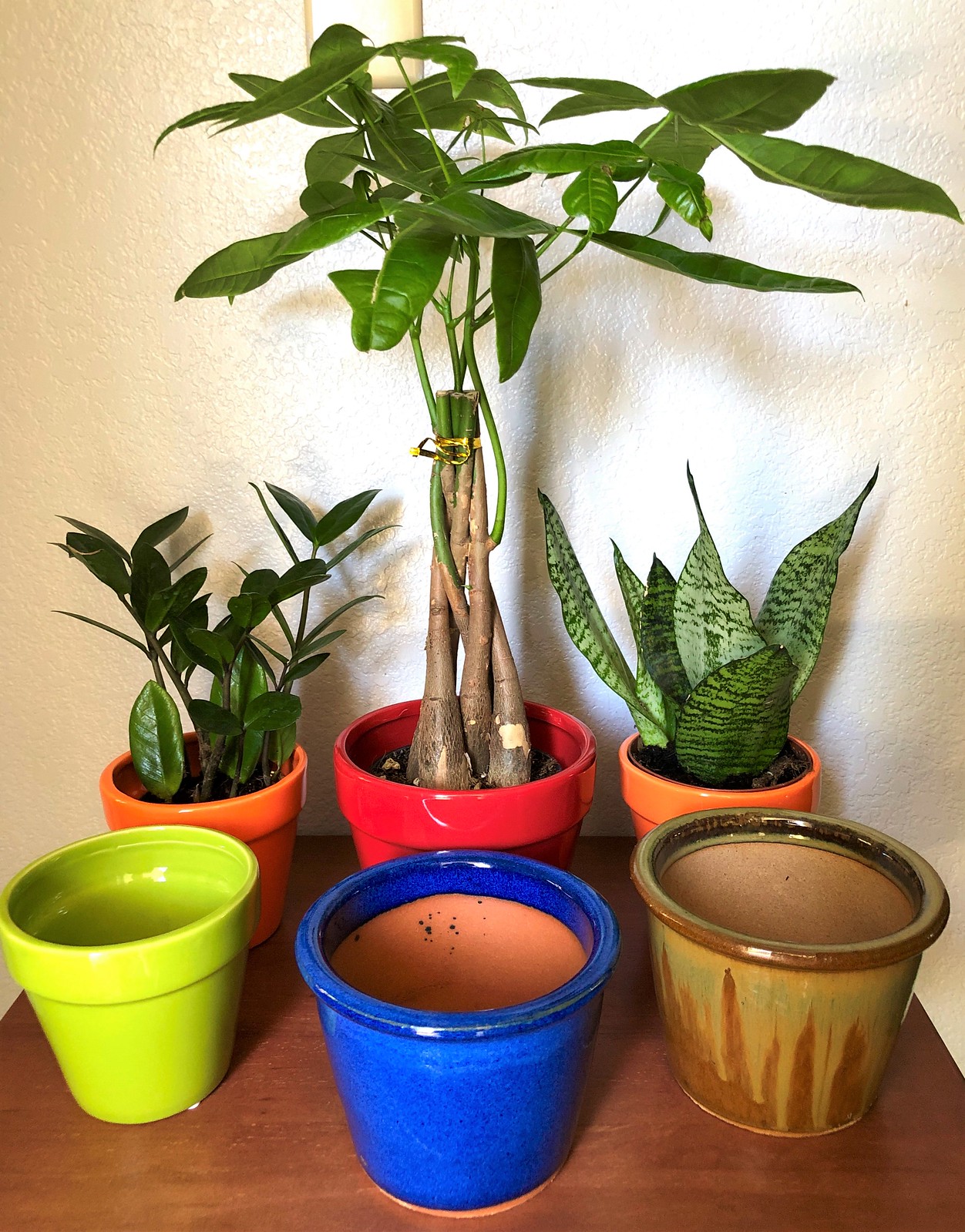In this photograph, a textured, rough-surfaced wall painted in a tan color forms the backdrop. The wall's uneven plaster adds a rustic charm to the scene. In front of the wall stands a dark brown wooden table, its rich wood grain providing a warm contrast. Arranged on the table are six flower pots. The back row features an orange pot with a plant bearing oval-shaped leaves, a red pot with a tall plant that has long leaves and a thick brown stem, and another orange pot with a plant that boasts sharp, pointy leaves. These pots are all filled with soil. The front row consists of three empty pots: a neon green pot on the left, a blue pot with an orange center in the middle, and a yellowish-brown pot with brown details on the right. The vibrant colors of the pots and the lush greenery of the plants infuse the scene with life and visual interest.